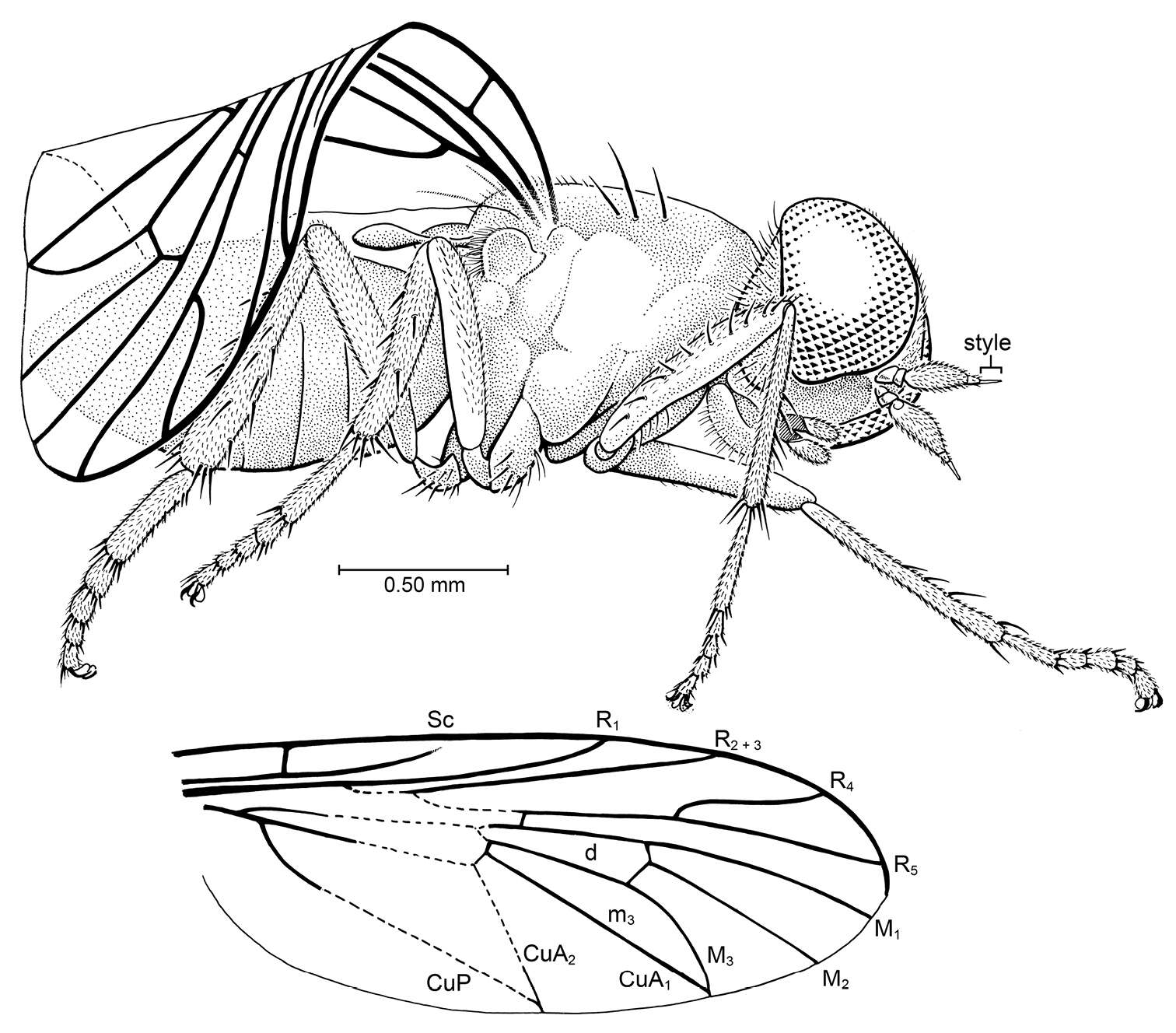This informational illustration represents a black and white anatomical drawing of a flying insect, possibly a bee or similar species. The primary image at the top shows the insect from a side view, oriented with its head to the right. Only the right side of its body is visible, including its elongated legs: two in the back, bent at the joints, and two in the front, with one extended forward and the other bent. Prominent features include its large, triangular-reflected eyes and sharp pincers extending from its head, labeled "Style." Emerging from its back are folded wings, and the body appears elongated with a rounded, oval shape tapering to a point at the rear. Below this primary image is a scale reference indicating 0.50mm. Additionally, a more detailed wing diagram is present at the bottom, marked with various letters and numbers like CUP, CUA, CUA1, SC, R1, R2+3, R4, R5, M1, M2, M3, delineating different segments and parts of the wing structure.